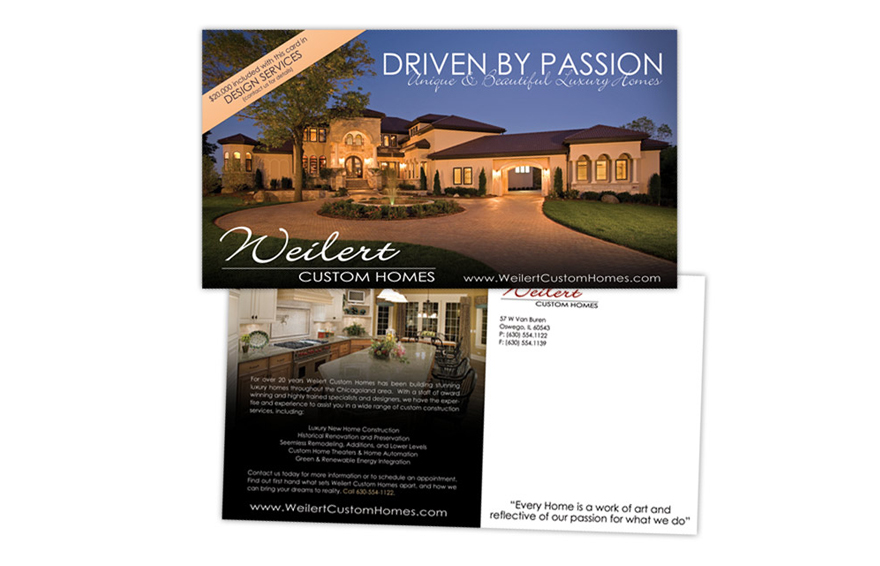The image displays a two-part advertisement for Weillert Custom Homes, consisting of two business cards. 

The top card prominently features the text "Driven by Passion" in large white font against the darkening backdrop of a dusk sky. Beneath this tagline, there is a picture of a grand luxury home with all its lights brightly shining, a spacious circular driveway, and a fountain in the center, symbolizing opulence and elegance. The home is portrayed against a setting sun, enhancing its aesthetic appeal. Additionally, a cream-colored stripe on this card reads "Weillert Custom Homes" along with the website address "www.weillertcustomhomes.com" and offers "$20,000 included with this card and design services" in smaller gray font.

Below this card, the second business card continues the advertisement theme, displaying a red cursive script spelling "Weillert" with "Custom Homes" written in gray beneath it. This card features an interior image of a well-appointed kitchen or dining room, showcasing the detailed and luxurious design elements offered by the company. Accompanying this image and text, the back of the card includes contact information and a motivational quote: "Every home is a work of art and reflective of our passion for what we do."

Together, these two cards present a cohesive and elegant advertisement for Weillert Custom Homes, emphasizing their dedication to creating luxurious and beautifully designed homes, driven by a passion for excellence in craftsmanship and design services.